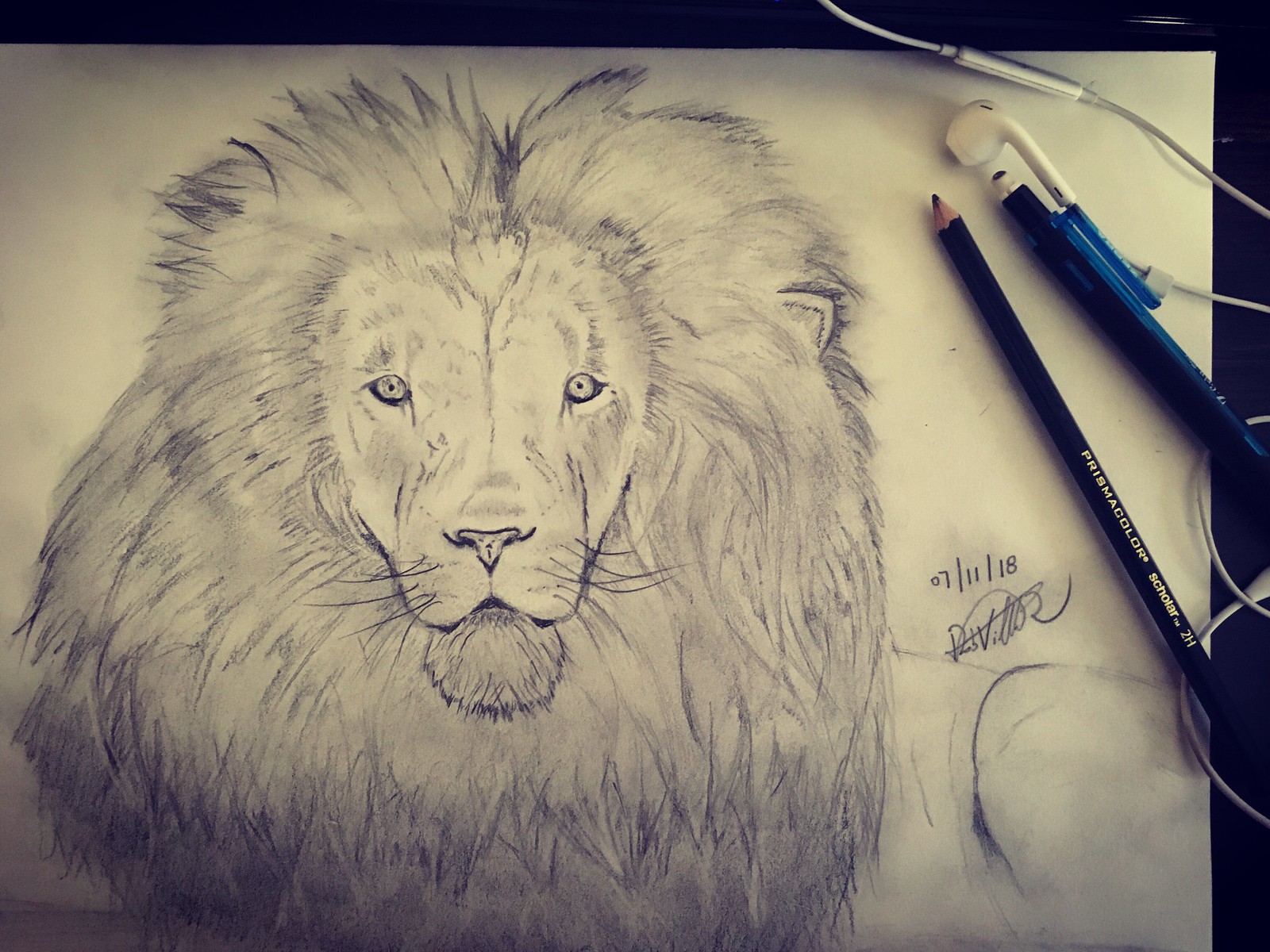In this black-and-white composition, a striking drawing of a male lion occupies the center of a large, pristine white sheet of paper. The lion, captured with detailed precision, gazes softly forward, his small eyes giving him a somewhat melancholic expression. His mane, while full and luxuriant at the bottom with distinctive tufts, is notably shorter on top than is typically seen. To the right of the drawing, the artist has carefully inscribed the date, 07-11-18, alongside an indecipherable signature.

Seen resting on the blank space to the right of the paper are the drawing implements: a Prismacolor Scholar 2H pencil and an eraser, along with a single earbud and its wire, casually placed atop the paper, hinting at the artist's creative process. The scene is set against a black surface with a barely perceptible dark background, focusing attention squarely on the artwork and the tools used to create it.